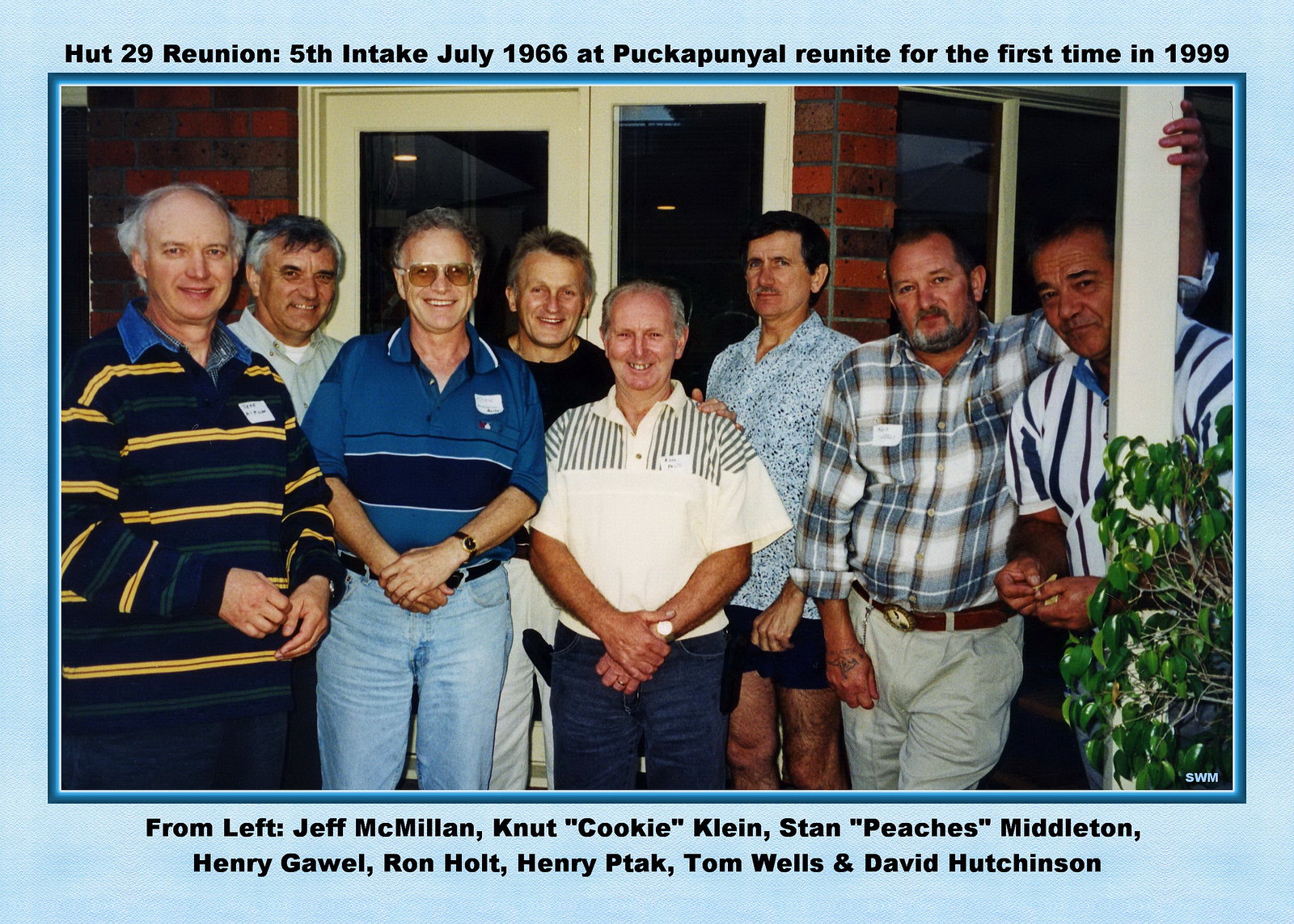The image shows a digitally framed photograph, bordered by a slightly darker light blue line within a light blue background. At the top of the frame, in black text, it reads: "HUT 29 Reunion, 5th Intake, July 1966, at Puckapunyal Reunite for the first time in 1999." The photo features a group of eight men, appearing to be in their late 50s or early 60s, dressed in casual attire and facing the camera. Each man has a white name tag on their chest. Below the photo, black lettering identifies them as (from left to right): Jeff McMillan, Knut "Cookie" Klein, Stan "Peaches" Middleton, Henry Gowell, Ron Holt, Henry Patak, Tom Wells, and David Hutchinson. They are standing in front of a red and gray brick building with white-framed glass doors, possibly sliding windows. A white rectangular post stretches from the bottom to the top on the right side of the image, and a small green shrub or plant is visible in the bottom right corner. The man on the far left is distinguishable by his polo shirt featuring horizontal yellow, blue, and green stripes.